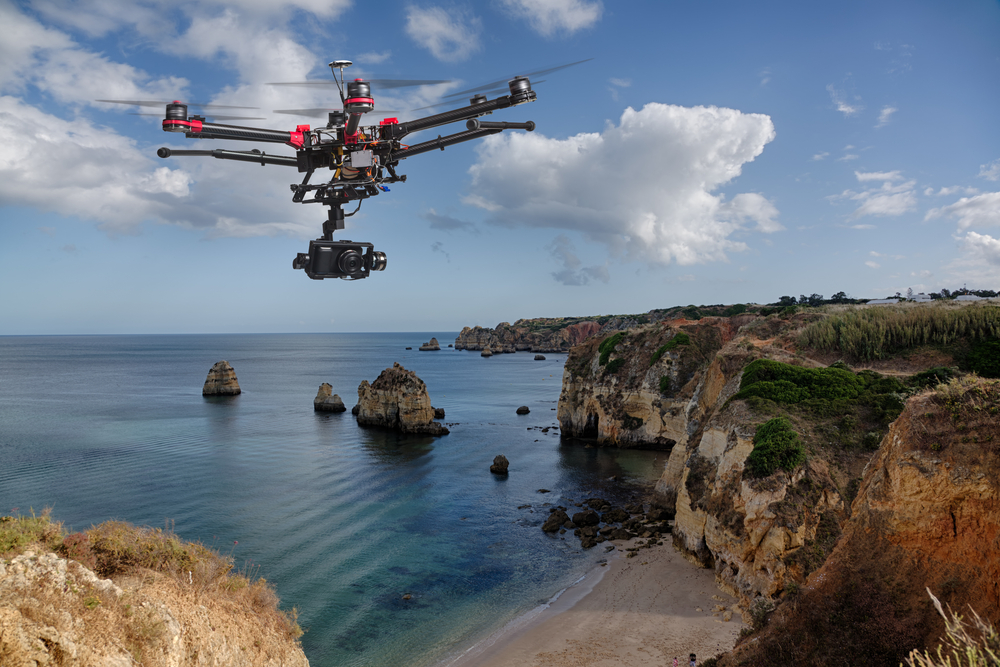A high-resolution photo captures a black hexacopter drone with six rotors, each equipped with red attachments at the front, soaring in the upper left corner of the image. The drone, equipped with a camera mounted on its underside and an antenna on top, is flying over a dramatic coastal ridge. Below, a serene beach stretches along the bottom edge of the image, merging into the gently wavy ocean observable on the left. The right side of the image reveals distant houses perched on verdant hills, with patches of vegetation dotting the landscape. The clear blue sky, adorned with scattered clouds, suggests the timing to be either late morning or early afternoon. The photo seemingly captures the perspective of the photographer standing on one of the cliff mounts, adding depth to the awe-inspiring coastal scenery.